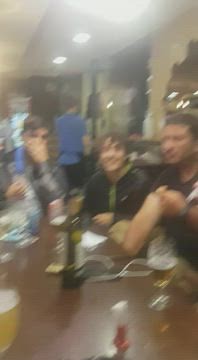This is a blurry photograph capturing a cozy, convivial scene of three men seated at a dark wooden table, which is strewn with various objects including beer glasses filled with amber liquid and a couple of bottles. The lighting in the image, consisting of recessed can lights and potentially a fluorescent light, creates a hazy, washed-out effect. The middle man is smiling warmly, while the person to his right stares into the distance and the individual to his left has their hand over their mouth, perhaps mid-laughter. Each man is dressed in darker attire - one in a dark shirt, one in a jacket, and the third in a mix of gray and blue. A female figure stands in the background with what appears to be a blue shirt and possibly an apron, suggesting she might be a waitress in a cozy establishment with hints of a kitchen area visible. The off-white walls are adorned with decorations, trimmed doorways are glimpsed, and there are dark-colored cabinets faintly seen in the blur. Despite the unclear details, the photograph radiates an overall ambiance of shared joy and camaraderie.